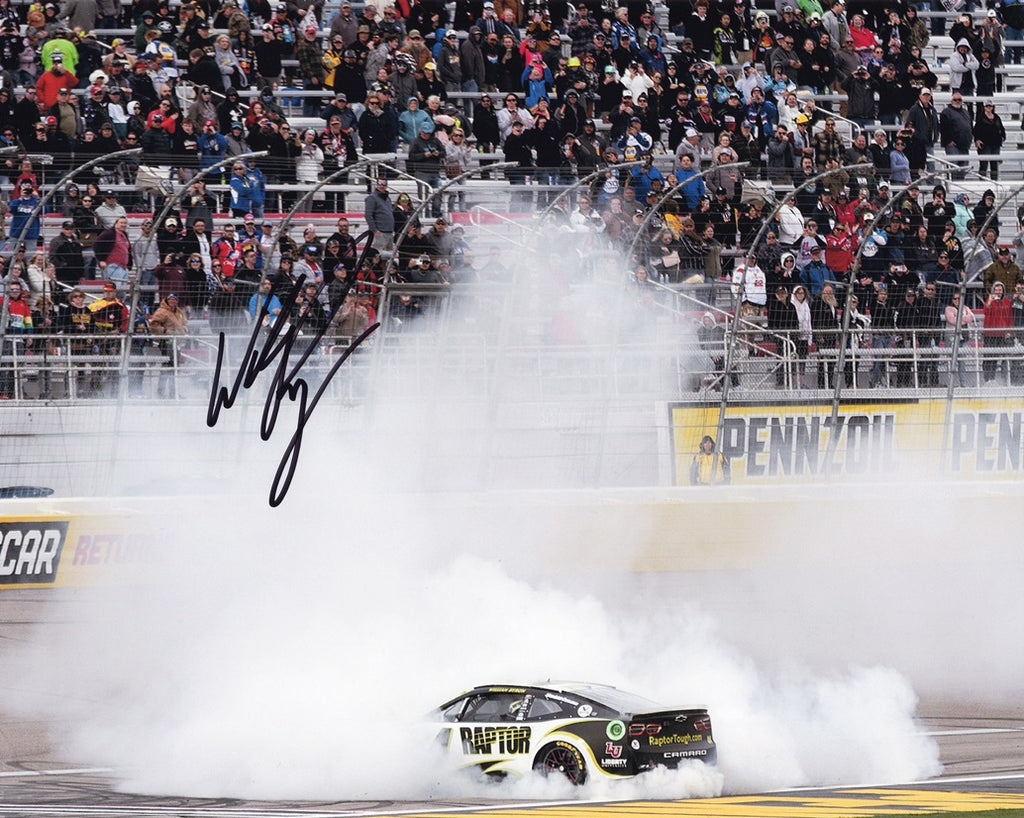A dynamic image captures a NASCAR race car dramatically smoking its tires, enveloped in a thick cloud of white smoke. The car, positioned centrally at the bottom of the frame, features a distinctive color scheme: a white door, a black top, and a black rear. Prominently displayed across the door, the word "Raptor" is emblazoned in bold black letters with yellow outlines. Near the back tire, a green circle, possibly the fuel cap, adds a splash of color. The rear of the car showcases a black bumper with "Camaro" written in white letters, topped by a yellow website URL "raptortuff.com" and decals of taillights crowned by a black Chevy emblem.

In the upper left corner of the image, a signature made with a black Sharpie is faintly visible. The background reveals a packed stadium with silver-colored seats, the audience standing attentively. A barrier featuring forward-sloping silver bars separates the racetrack from the spectators. On the right side of the image, a yellow Pennzoil banner with black lettering is visible, beside which stands a woman in a yellow jacket. This vivid scene captures both the intensity of the race and the electrifying atmosphere of the crowd.